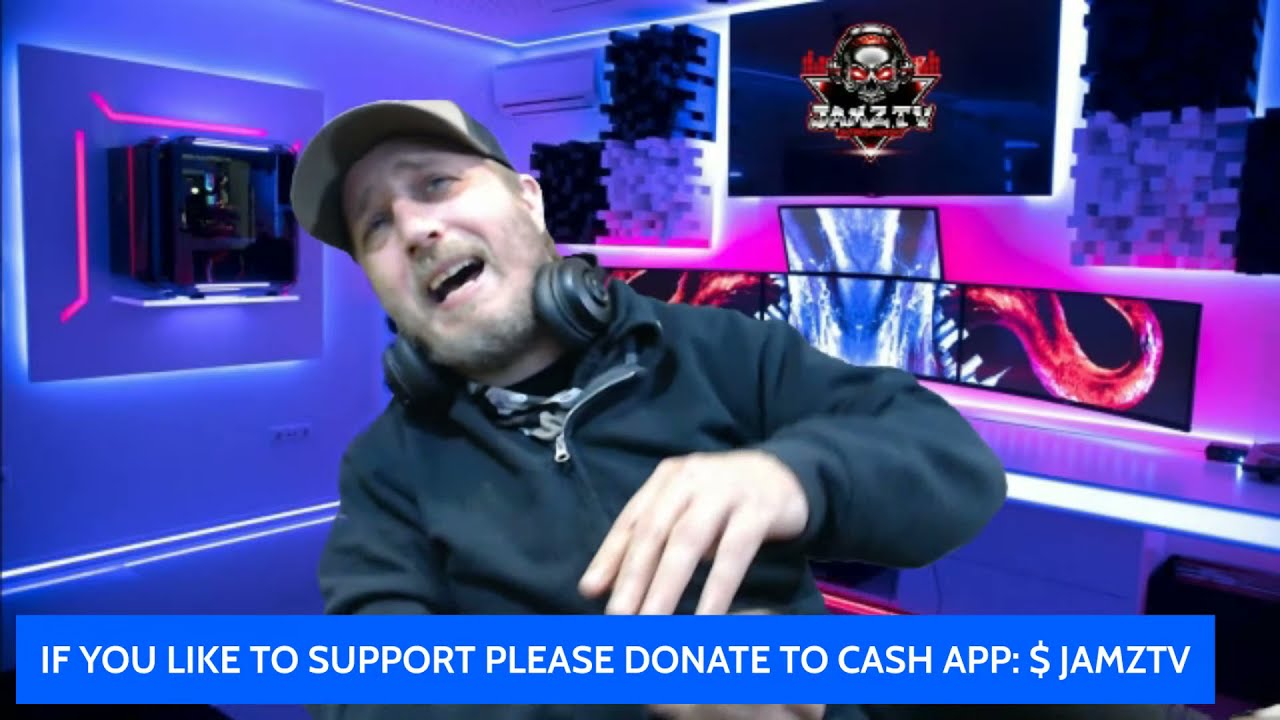The image depicts a screenshot of a live stream session from a platform named JAMZ TV. The bottom of the screen features a blue rectangular box with white, capitalized, sans-serif text that reads, "If you'd like to support, please donate to Cash App: $JAMZTV." In the foreground, a man with a light brown beard is wearing a green cap with a white front and a green back. He has black headphones around his neck and is dressed in a black zip-up sweatshirt with a dark t-shirt underneath. His expression appears pained or distressed, and his head is tilted to the right. His left arm is raised to chest level, with his palm facing downward. The background suggests a computer gaming room, adorned with neon blue, pink, and purple lighting. Numerous computer monitors, approximately five, and a TV are visible, with digital graphics and pixelated designs. Prominent is a graphic with "JAMZ TV" and an icon resembling a triangle with a skull and red and black designs.